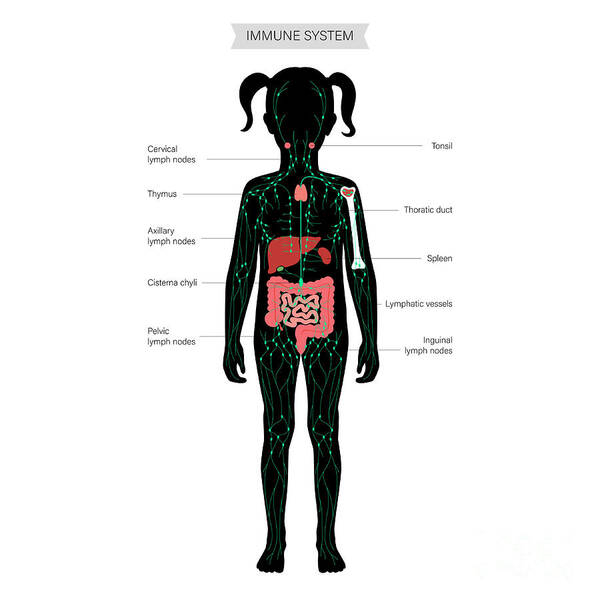This vertically aligned rectangular image serves an educational purpose by illustrating a young girl's immune system. The image is a black silhouette of a girl with pigtails, indicating she is likely around five years old. Within the silhouette, various organs and lymph nodes are meticulously labeled. Notably, there are bright green dots representing different lymph nodes scattered throughout the body, and specific organs are highlighted.

In the upper part of the image, a gray banner with the words "IMMUNE SYSTEM" in bold black print provides context. On both the left and right sides of the silhouette, labels point to different parts of the girl's body: 

- On the left, the labels read cervical lymph nodes, thymus, axillary lymph nodes, cisterna chyli, and pelvic lymph nodes.
- On the right, the labels identify tonsils, thoracic duct, spleen, lymphatic vessels, and inguinal lymph nodes.

Highlighted organs include the intestines, shown in pink at the bottom, and an outlined white bone in her upper arm. The face lacks detailed features but includes green curved lines on each side with two pink dots near the chin, indicating lymph nodes. This detailed diagram is designed to educate viewers, such as parents or medical students, on the human lymphatic system using the young girl's silhouette as a reference.